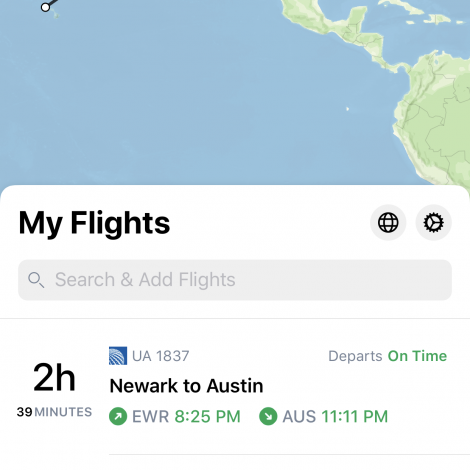This image depicts a smartphone screen showing flight details. The top portion of the screen displays a map, predominantly covered by blue waterways, likely oceans, with some land visible from the upper right to the lower right corner. Centered at the top in bold, black text is the title "My Flights" accompanied by a globe icon and a clock symbol.

Below the heading, there is a search bar with a magnifying glass icon labeled "Search and add flights." Directly underneath, a time duration of "2 hours 39 minutes" is noted, indicating the length of the flight.

The flight details for UA 1837 from Newark (EWR) to Austin (AUS) are displayed next. The text "UA 1837, Newark to Austin" is printed in black, and there's a status note reading "Departs on time" in green. The specific departure and arrival times are also provided: Newark departure at 8:25 p.m. (EWR 825 p.m.) and Austin arrival at 11:11 p.m. (AUS 11 11 p.m.), both times highlighted in green to likely indicate timeliness.